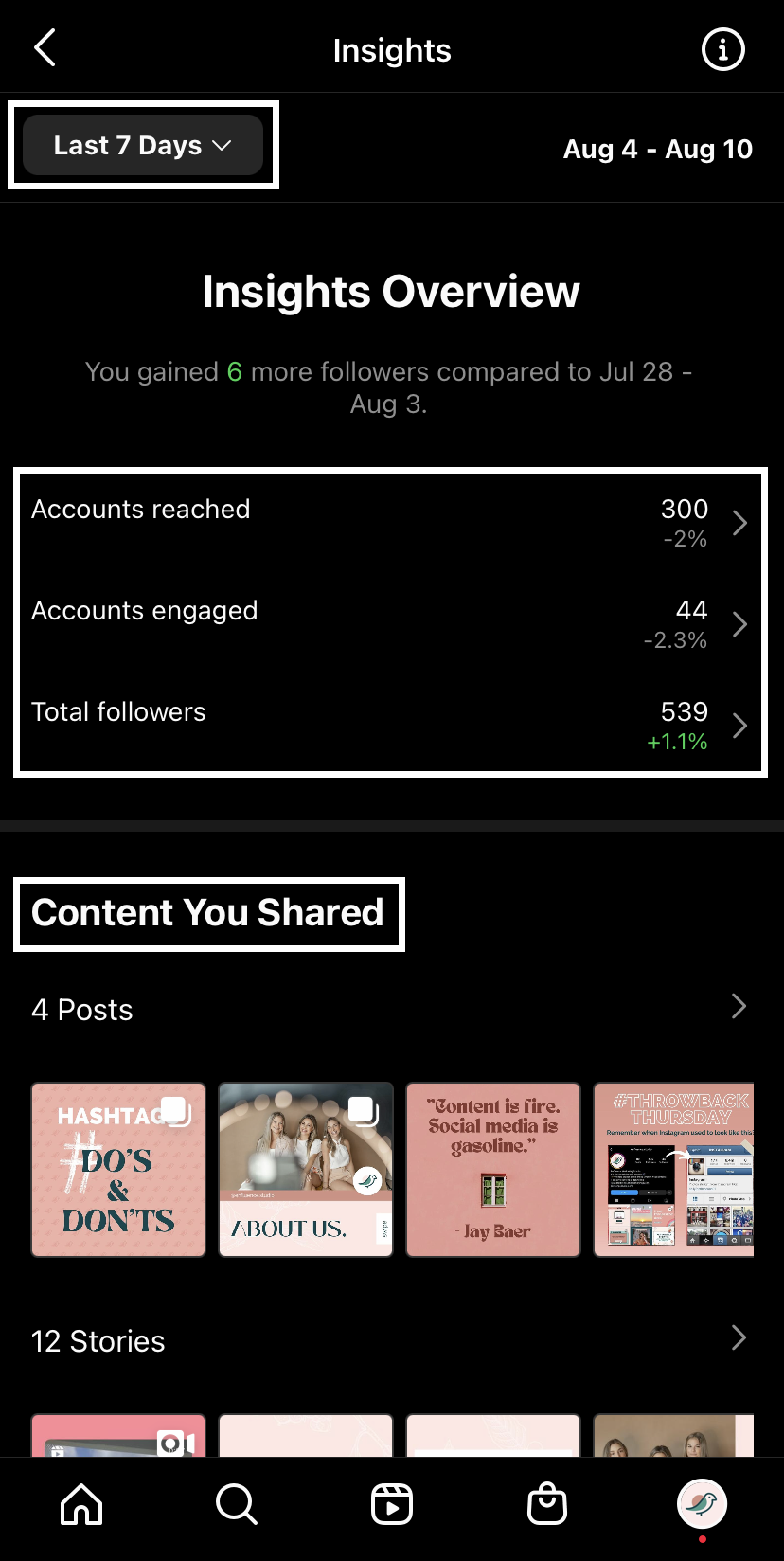This screenshot captures the Insights page of a social media analytics dashboard. At the top, the title "Insights" is prominently displayed with a date range selector set to "Last 7 Days," specifically from August 4th to August 10th. Below the date range, an "Insights Overview" summarizes that the account gained six more followers compared to the previous week (July 28th to August 3rd). 

Key metrics are detailed as follows:
- **Accounts Reached:** 300, a decrease of 2%.
- **Accounts Engaged:** 44, a decrease of 2.3%.
- **Total Followers:** 539, an increase of 1.1%.

The content shared during this period includes posts titled "Hashtag Do's and Don'ts," "About Us Content is Fire, Social Media is Gasoline," and a segment for "Throwback Thursday," along with 12 stories.

The user interface resembles that of a social media application, likely TikTok, based on the layout and icons. At the bottom, there are navigation buttons, including a Home button, a Search button, a Bag button (possibly for shopping), and a profile icon on the far bottom-right. Despite the slight decreases in reach and engagement, the account has seen a modest increase in followers.